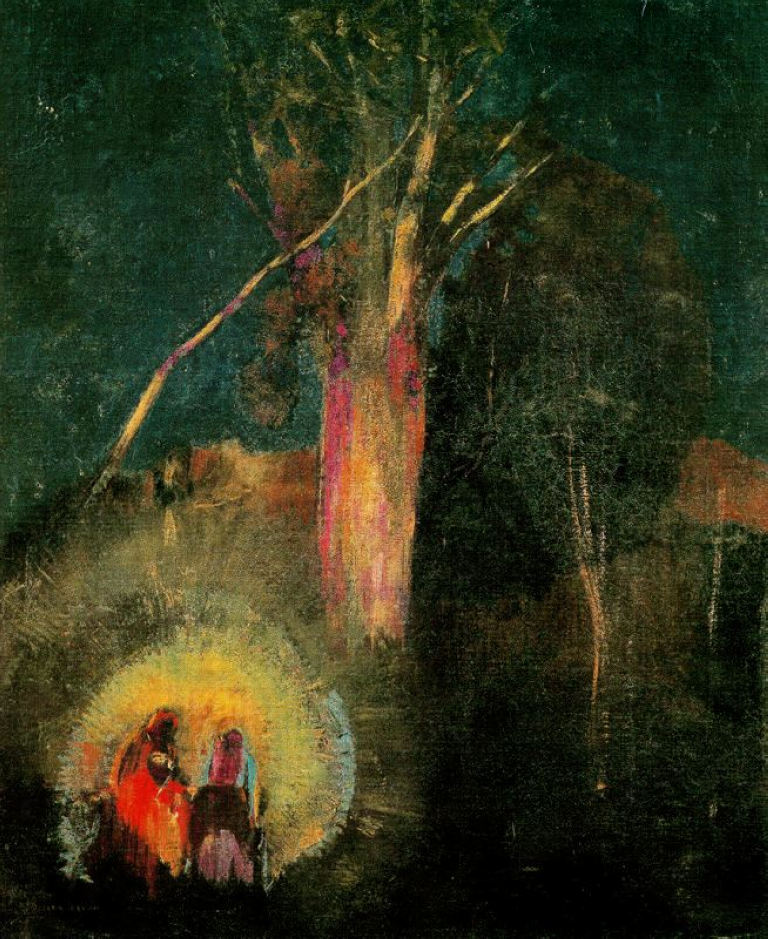This painting captures a nighttime scene with rich, dark colors. Dominating the image is a large, multi-colored tree with a trunk in hues of reds, pinks, yellow, and white that extends into branches painted in yellowish and darker green tones. The tree stands tall, reaching into a deep, greenish, dark blue sky. To the right of this imposing tree, a forest of darker trees and shrubs can be seen, adding depth to the scene.

In the lower left corner, within a bubble-like, circular glowing light, are two small, humanoid figures. The figure on the left appears to be male, wearing a flowing orange robe that covers his body. The figure on the right is less distinct but seems to be dressed in black pants and a blue shirt or possibly a light blue veil that drapes over the head and body. These characters are seen from the back, gazing at the illuminated tree in front of them. A dark strip runs along the bottom edge of the painting, grounding the scene.